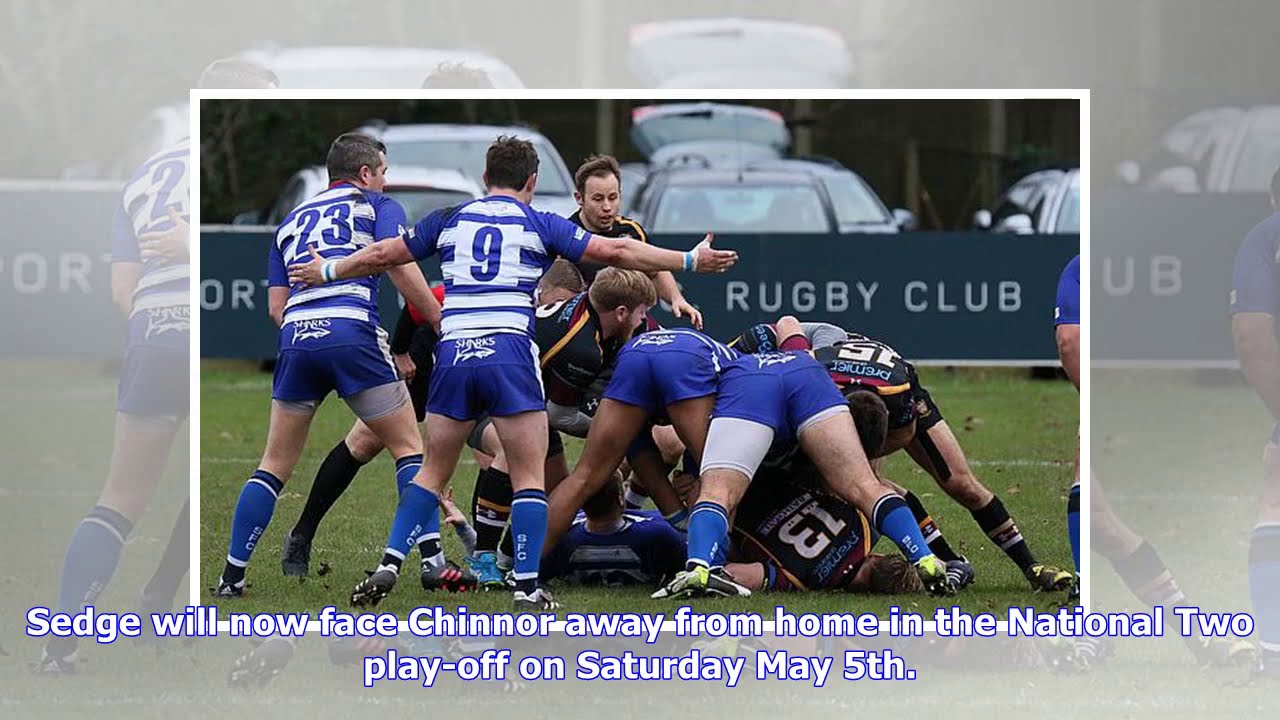The image portrays an intense rugby match on a green grass field. Two teams are competing: one team, the Sharks, donned in royal blue and white striped jerseys and blue socks, and another team wearing black jerseys with yellow stripes and red accents. Key players from the Sharks include numbers 9 and 23, both with short hair and blue shorts, and numbers 13 and 15 on the opposing team. The scene captures a heated moment as the players are piled up in a scrum, striving for control of the ball. In the background, there's teal signage that reads "Rugby Club," along with some parked cars, one with its trunk open. The image is bordered in white, with a blue-bordered white caption at the bottom, reading: "Sedgwil now face Chinor away from home in the National 2 playoff on Saturday, May 5th." The photograph is set under an overcast sky, suggesting it was taken during midday.